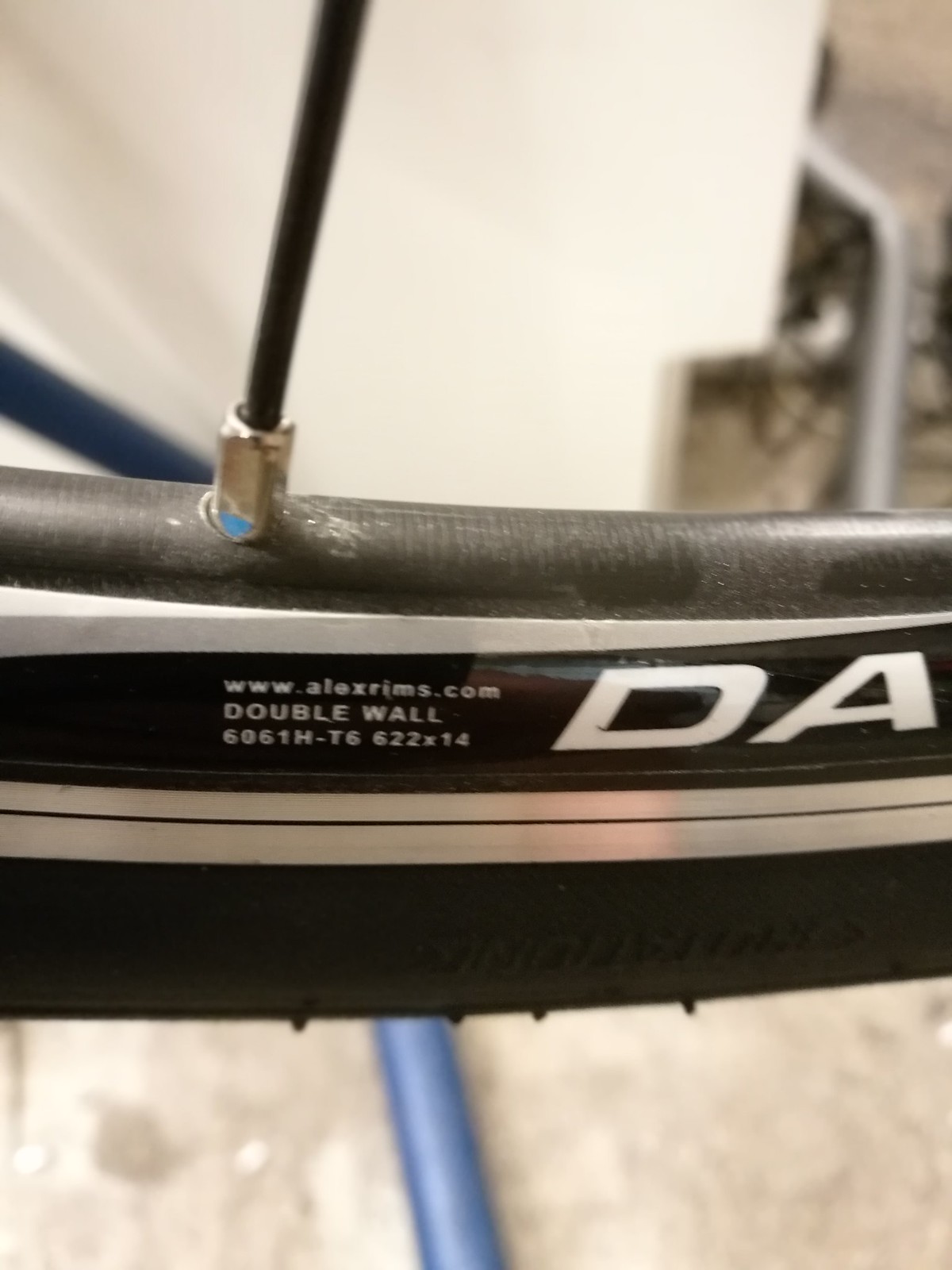A close-up, tall rectangular photograph focuses on a black bicycle wheel, extending horizontally just below the center of the frame. The wheel features two white stripes and prominent white text that reads "www.alexrims.com" along with "double wall" and "6061H-T6 622 x 14." Adjacent to this text are large capital letters "D" and "A." Above the wheel, there's a curved metal pole connected to a black wire via a gold screw. The background reveals a large white object and a gray metal pole on the upper right, with a light brown, possibly concrete, floor beneath. Some blue hose runs vertically towards the top left of the image, adding to the industrial feel of the scene.